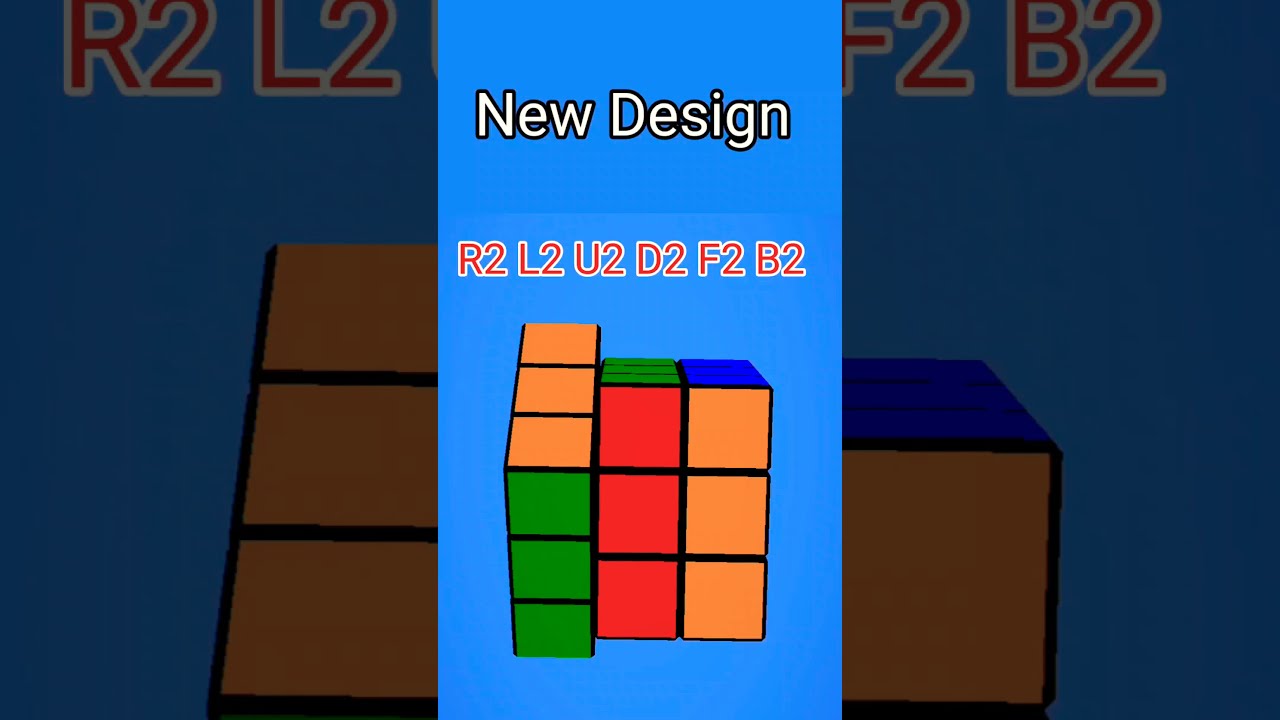The image features a bright blue background with a central section that is light and emphasized, while the left and right sections are tinted and show zoomed-in portions of the central image. At the top of the center section, "New Design" is written in white text with a black outline. Below this, in red text with white outlines, it says R2, L2, U2, D2, F2, and B2. Underneath this text, there is a Rubik's Cube. Looking straight at the cube, the right column has orange squares, the center column has red squares with a barely visible green square on top, and the left column is slightly tilted upwards showing orange on top and green on the bottom. The right zoom shows a close-up of the F2 and B2 letters, while the left zoom showcases the R2 and L2 letters along with part of the Rubik's Cube. The slightly darker and tinted background suggests a possible digital design or mock-up, perhaps intended for a mobile phone display.